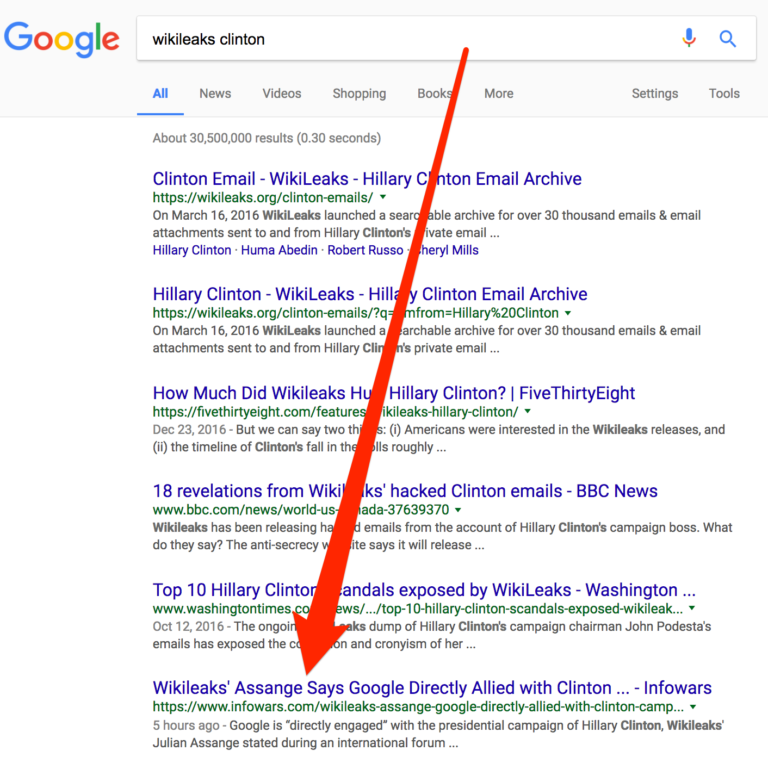Detailed Caption: 
The image is a screenshot of a Google search results page captured on a computer screen, characterized by a clean, white background at the top. The upper left corner features an off-white rectangle displaying the iconic Google logo, composed of the word "Google" rendered in primary colors - blue, red, yellow, and green.

To the right of the logo sits the search field, within which the query "WikiLeaks Clinton" has been typed. Adjacent to the search field on its right side are two small icons: a blue microphone symbol for voice command and a magnifying glass icon representing the search function.

Directly below the search field, a navigation bar presents various search options: "All," "News," "Videos," "Shopping," "Books," "More," "Settings," and "Tools," with the "All" option currently selected.

A conspicuous, photoshopped red arrow extends vertically from the search field down to the bottom search result, suggesting the importance of the highlighted content.

The bottom search result, notable for the font color and the source, is styled in blue text and reads: "WikiLeaks Assange says Google directly allied with Clinton... InfoWars." This link is followed by the web address: "https://www.infowars.com."

InfoWars, a controversial website known for its conspiracy theories and sensationalist content, is implied to have provided the search result mentioned.